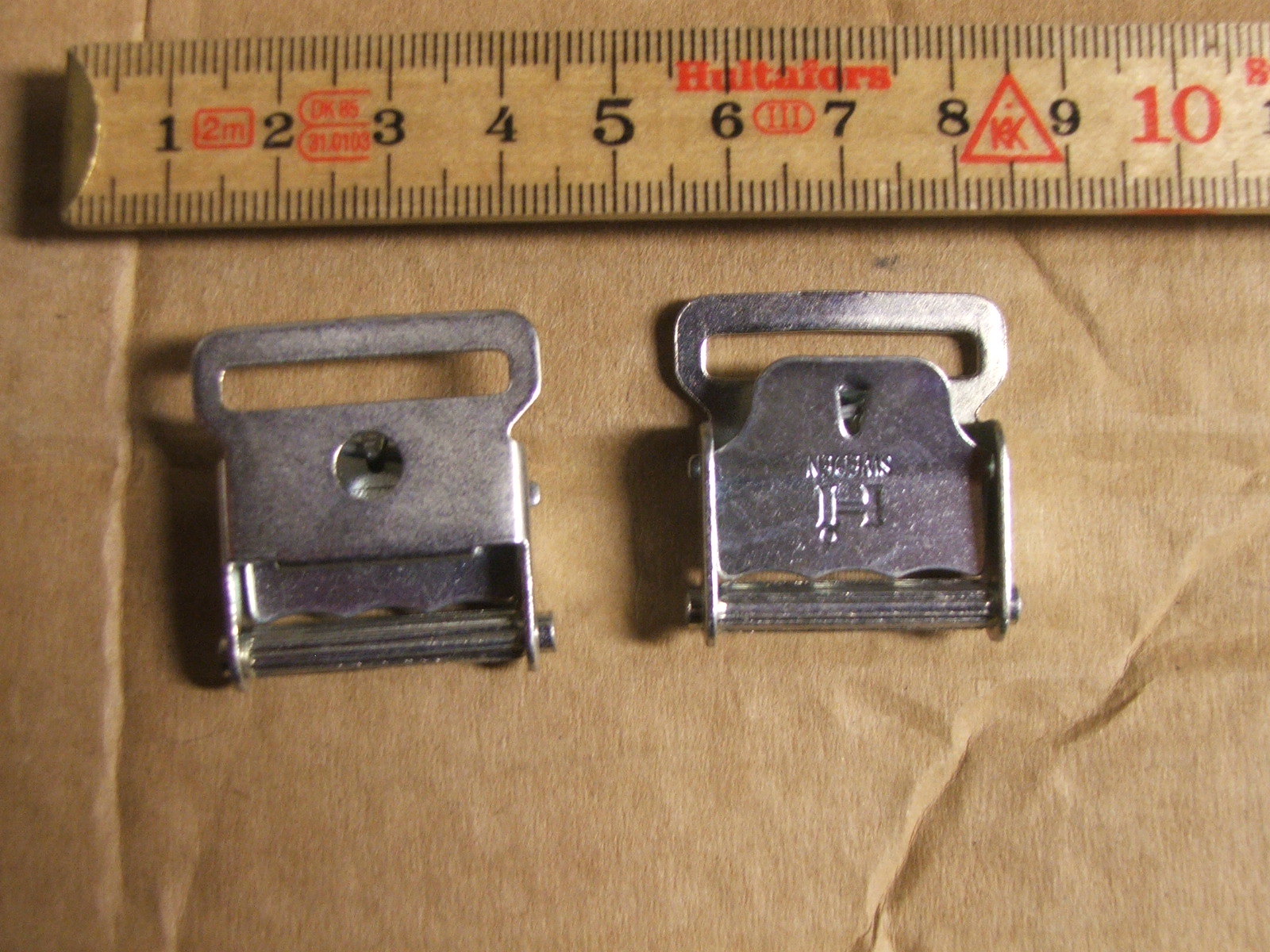This image features two silver belt buckles displayed on a piece of light brown, possibly creased, paper or cardboard. The buckle on the left is positioned frontwards, while the one on the right faces backwards and has an engraved "H" on its back. Above the buckles is a wooden ruler marked in centimeters, showing measurements up to 10.8 cm. The ruler, which is sandy-colored, has distinct red and black printed elements: between the 6 and 7 cm marks, the phrase "HALT SEPHORA" appears in red text. A red triangle enclosing "KK" is situated between the 8 and 9 cm marks. The 10 cm mark is also highlighted in red. Additionally, there is a red-cornered rectangle with "2M" between the 1 and 2 cm positions. Two circles containing the inscriptions "DK85" and "31.0103" are found between the 2 and 3 cm marks. The detailed arrangement and various markings on the ruler contribute to the unique composition of the image.